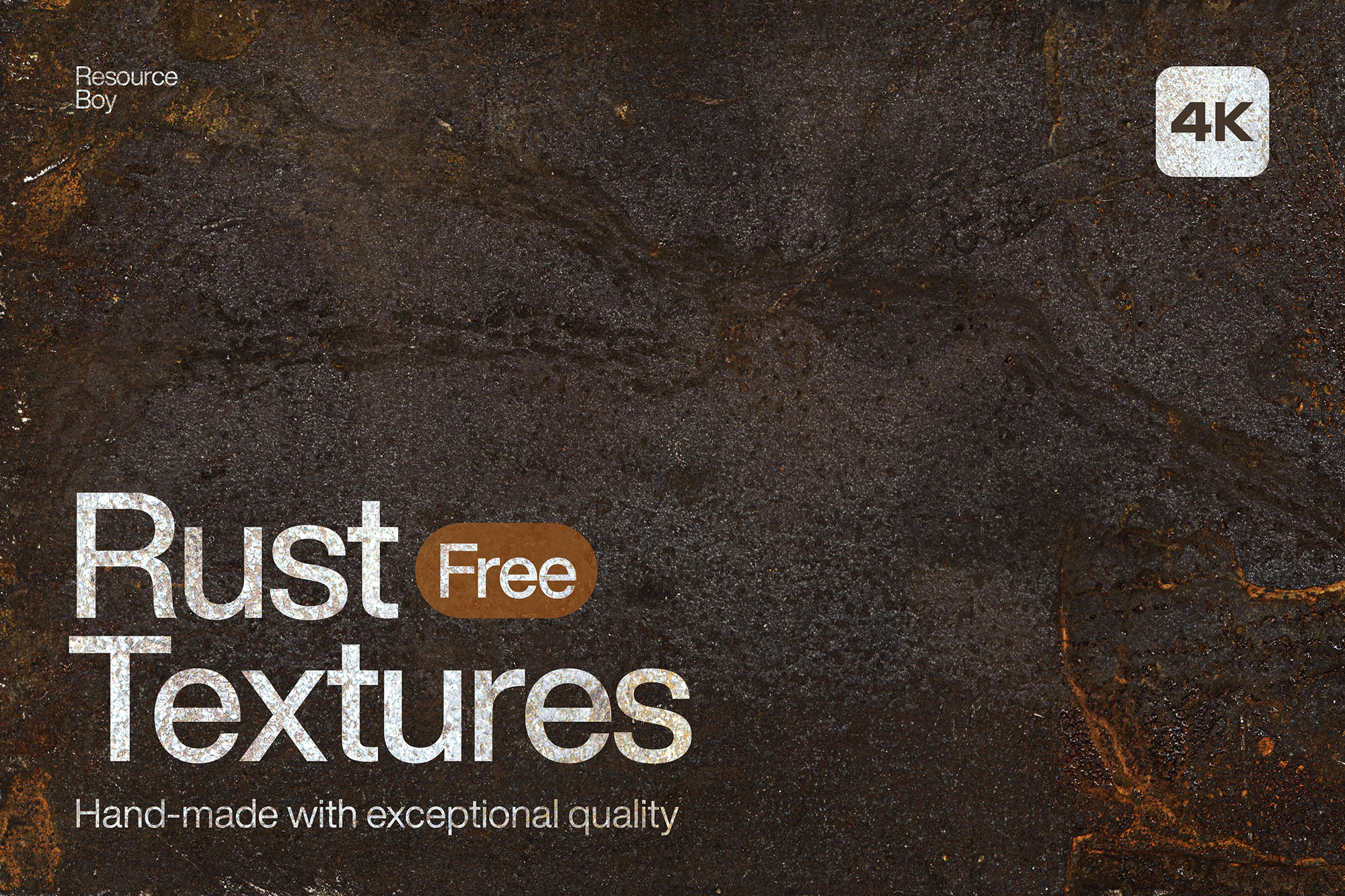A captivating image showcases a rich paint texture set against a black backdrop speckled with brown and white flecks. In the upper right corner, a white square bears the brown printed text "4K," adding a touch of high definition appeal. The lower left corner contains white text that reads "Resource Boy" and further details, "Rust-free textures, handmade with exceptional quality." The paint color displayed has a unique, marbled effect reminiscent of stone or granite, with veins of lighter colors, particularly emphasized in the lower right corner. This image highlights not only the aesthetic appeal of the paint but also its durability, emphasizing its rust-resistant qualities.